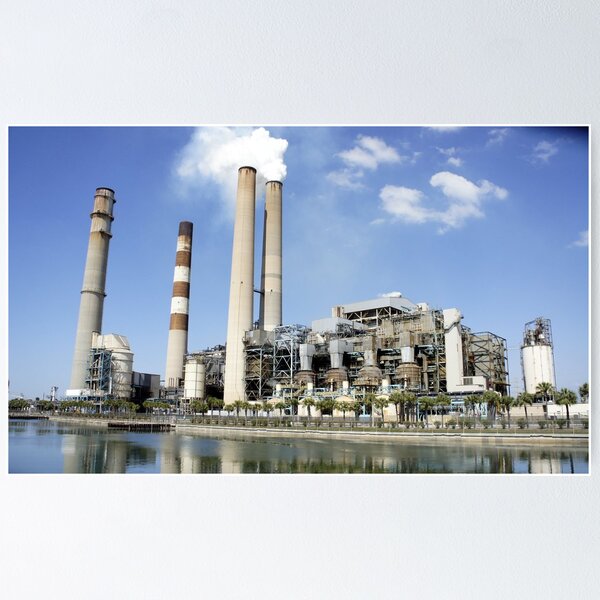The image depicts a large industrial factory or production plant situated along the edge of a waterway, which could be a canal or a man-made lake. The facility is characterized by its dull colors of metal and concrete, giving it a somewhat unexciting and utilitarian appearance. Prominent in the scene are four giant smokestacks, with white smoke emerging from one or two of them and blending into the white clouds against a bright blue sky. The entire structure, composed of extensive metal scaffolding and several stories high, dominates the landscape. Along the water's edge, a row of green-leaved trees, resembling palm trees, creates a natural barrier between the factory and the water, adding a touch of greenery to the industrial setting. The reflection of the factory and the trees is clearly visible in the calm water.